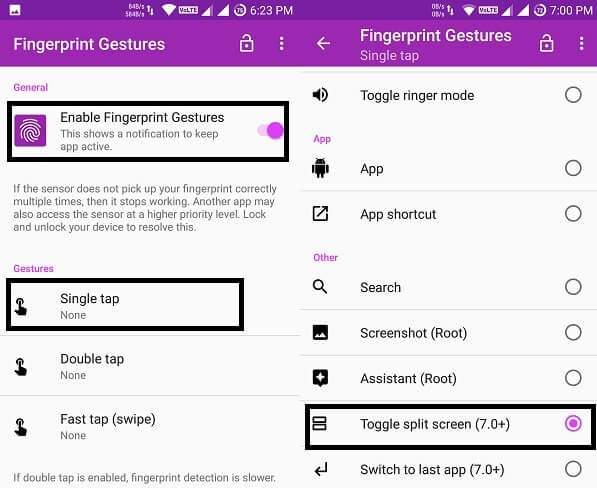The image, displayed on a smartphone screen, is divided into two sections. The top section features a pink background with white text that reads "Fingerprint Gestures."

On the left side, within this top section, there's another portion with a white background. The heading "General" is written in pink at the top. Below it, the text "Enabled fingerprint gestures" is also in pink, indicating a notification that keeps the app active. Accompanied by a pink toggle switch, which is turned on, this part is outlined with a black box. Below this, additional information states: "If the sensor does not pick up your fingerprint correctly multiple times, it stops working. Another app may also access the sensor at a higher priority level. Lock and unlock your device to resolve this."

Further down, still on the left side, the text "Gestures" appears in pink. There are three gesture options listed: "Single Tap," "Double Tap," and "Fast Tap or Swipe," all with the status "None." The first option, "Single Tap," is outlined with a black square. At the bottom of this section, there is a note in pink text: "If double tap is enabled, fingerprint detection is low."

On the right side of the image, following the selection of "Single Tap," options related to this gesture are displayed. The heading "Fingerprint gesture: Single tap" is followed by several toggle options, all of which are turned off except for "Toggle split screen (7+)." Each option is presented as follows:
- Toggle: Ringer mode (not on)
- App (not on)
- App shortcut (not on)
- Search (not on)
- Screenshot, root (not on)
- Assistant, root (not on)
- Toggle split screen (7+), with a black outline indicating it's on
- Switch to last app (not on)